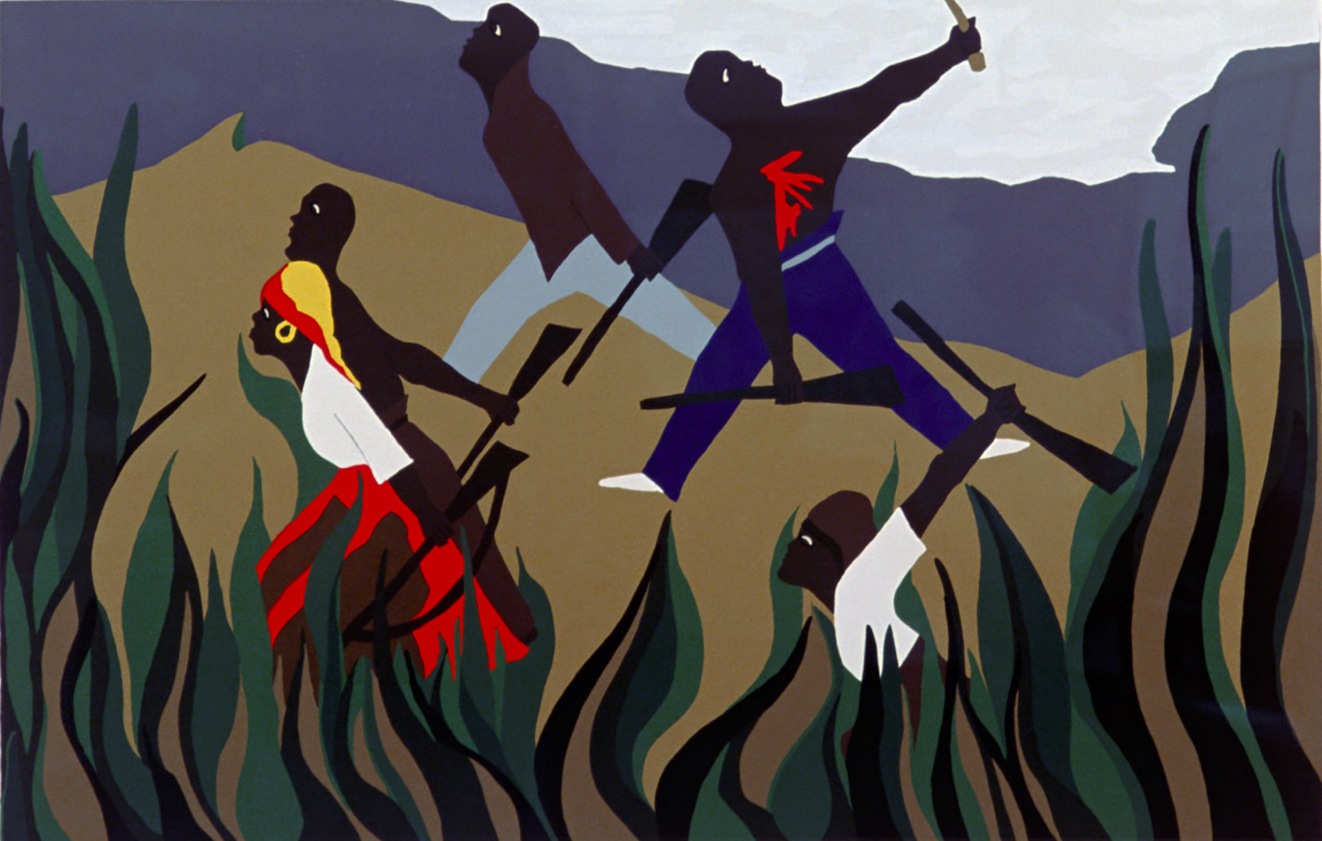The image is a highly detailed graphic illustration in a traditional African style, showcasing five black individuals standing and holding guns. The figures are arranged in a circle and appear to be standing amidst tall, flowing, olive green and black vegetation that resembles long grass. The ground beneath them is an unadorned matte tan color. The background features layers of slate blue transitioning into white, suggesting the sky and clouds, with some areas appearing reminiscent of mountains.

Central in the group is a woman adorned with a yellow headscarf accented in red and orange, a bright yellow hoop earring, a white shirt, and a vivid red skirt. To her left, a man with blue pants, no shirt, and white socks stands, holding both a gun and a knife, with a noticeable red spray on his upper chest as if he has been shot. Another man, bare-chested in light blue pants and carrying a long gun, walks beside a woman. Other notable details include a man wearing a brown shirt and light-colored pants and another figure, possibly a child, holding a gun raised in the air while dressed in a white shirt.

This vibrant scene captures the intense emotions of the subjects, set against an evocative backdrop of contrasting colors and textures in the sky, ground, and surrounding foliage.